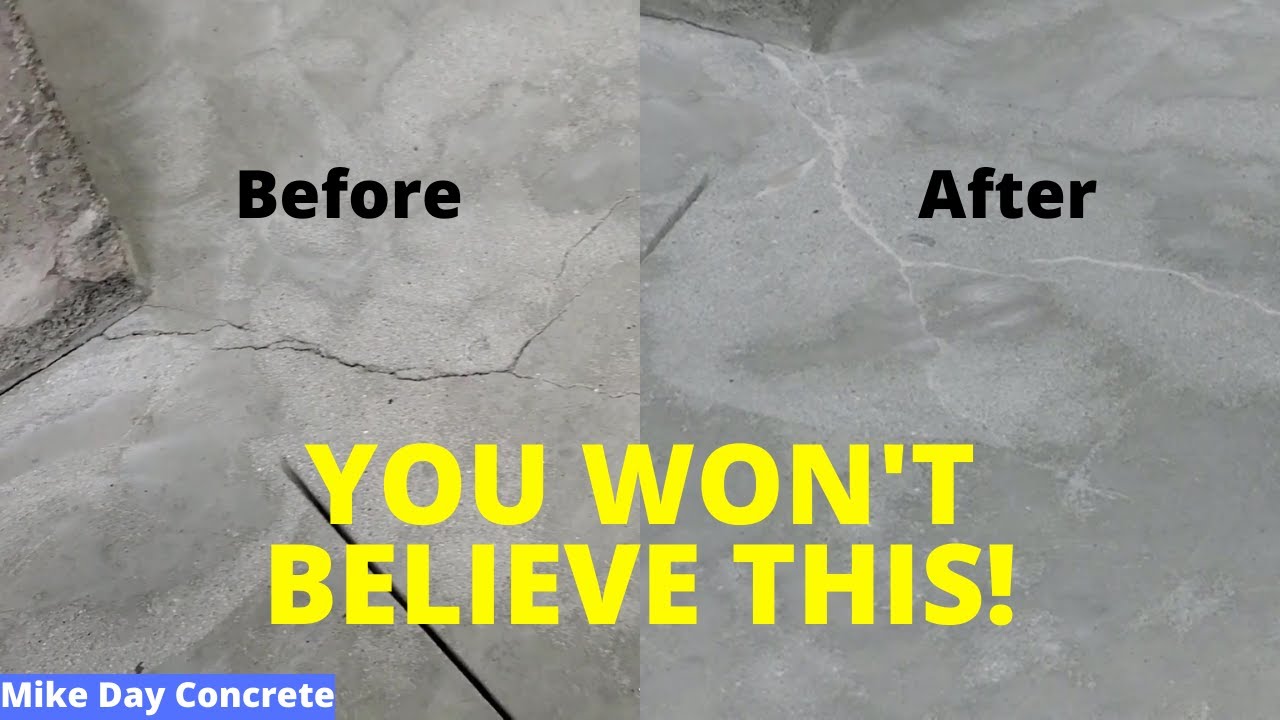The photograph serves as a detailed before-and-after comparison demonstrative ad for concrete repair by Mike Day. On the left side, the image showcases an old piece of concrete riddled with noticeable but not massive cracks, labeled "BEFORE" in black lettering. The right side presents the same concrete after repair, with the cracks filled in using a lighter gray adhesive or bonder, visibly smoother yet discernible, labeled "AFTER" in black font. The background to the text on the left is cracked concrete while the right shows the repaired state from a slightly different angle, illustrating the transformation. Dominating the foreground in bold, large yellow block letters are the words "YOU WON'T BELIEVE THIS!" At the bottom left-hand corner, within a horizontal blue bar, "Mike Day Concrete" is inscribed in crisp white lettering, signifying the person responsible for the repair work and emphasizing his capability in fixing concrete imperfections effectively.